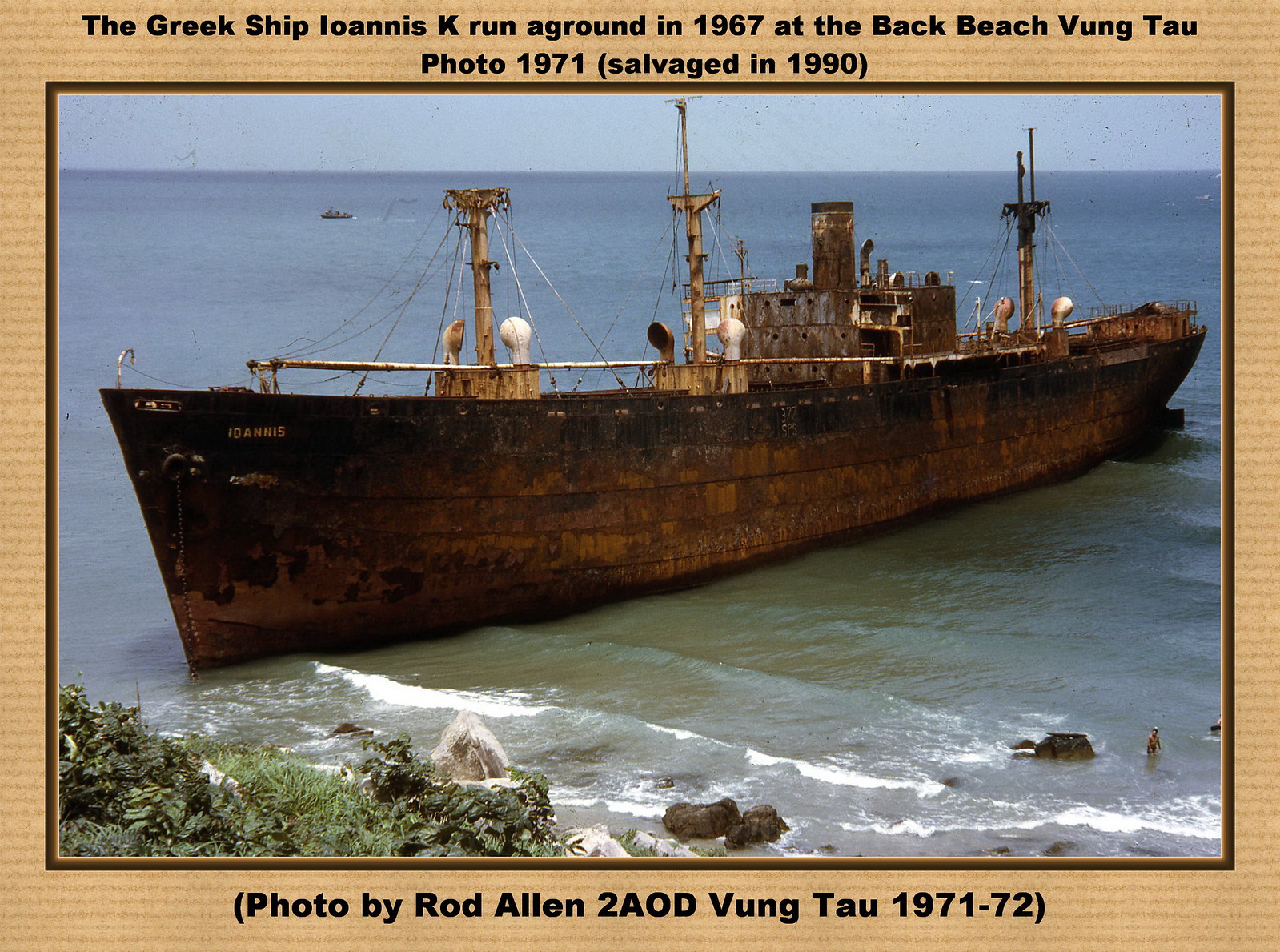The image depicts the rusted and worn-out Greek cargo ship "Ioannis K" that ran aground in 1967 at Back Beach, Vung Tau, captured in a professionally taken photo in 1971 by Rod Allen during his time with AOD Vung Tau from 1971 to 72. Salvaged in 1990, the ship, displaying a copper-colored rust, sits partially in the water with its bow embedded in the sand. The sky above is a clear blue with no clouds, and the sea in the background is a grayish-blue with small waves hitting the shore. To the left corner, near some green vegetation and rocks, a tiny figure, possibly a person, can be seen near the water around 300 feet away from the ship. The image has a black border with a thicker tan-beige outer border, and features black text above and below providing historical context.